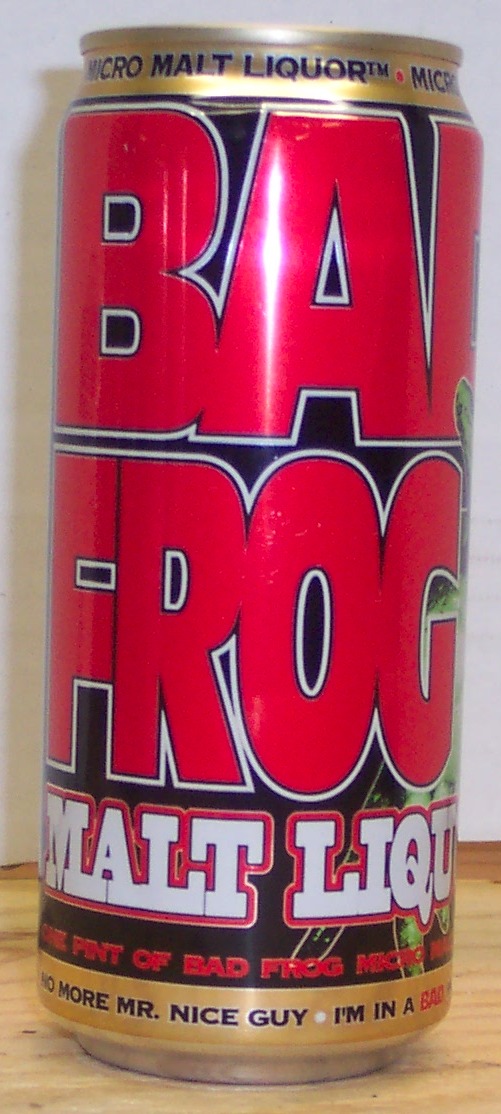This close-up photograph features a tall, gold can of micro malt liquor labeled "Bad Frog." The can prominently displays large red letters that spell "Bad Frog" across a black banner, occupying roughly 75-80% of the can's surface. Each red letter is outlined in white, making the bold text stand out. Below this, in white letters outlined in red, the words "Malt Liquor" are clearly visible. Further down, a tagline in black lettering states, "No More Mr. Nice Guy. I'm in a bad...," though the final word is obscured. The can appears very cold, with visible condensation, and is placed on a light blonde wooden table, against a white background.